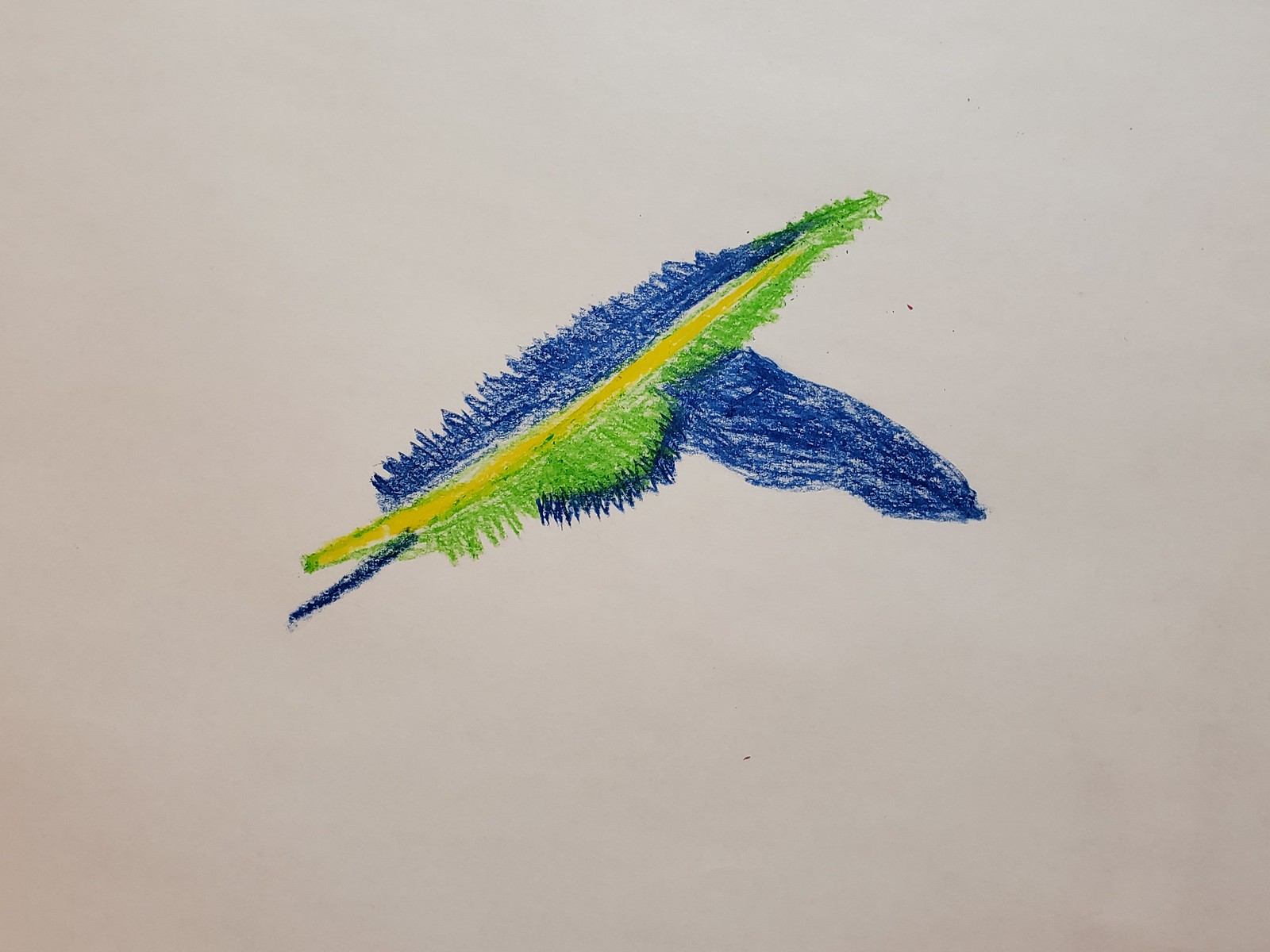This image features a detailed crayon drawing on a wrinkled, white piece of paper that appears light gray due to surrounding shadows. At the center, there are two feather-like shapes arranged diagonally. The feather on top has a prominent yellow stem running upward, adorned with green zigzag patterns towards the right and top. The left side of this feather-like shape features darker blue shading, transitioning to lighter blue in a jagged, triangular section. Beneath it, about midway up, lies a horizontally positioned blue feather, defined by dark blue wisps to denote its form. The overall composition is vibrant, combining elements of yellow, green, and blue against the subtle backdrop of the paper.